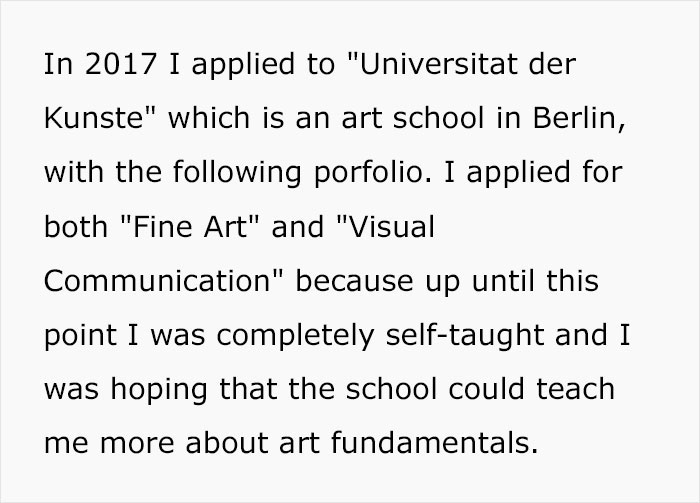The image features a paragraph of black text on a very light gray background, enclosed within a thin, slightly darker gray hairline border. The font is a traditional serif style, resembling Times New Roman, large, well-spaced, and easy to read. The text reads: "In 2017, I applied to Universität der Kunst, which is an art school in Berlin, with the following portfolio. I applied for both fine art and visual communication because up until this point, I was completely self-taught, and I was hoping that the school could teach me more about art fundamentals." The text, organized into eight lines without full justification, occupies most of the rectangular space, with some margin around the edges. There are no other elements or designs present in the image.